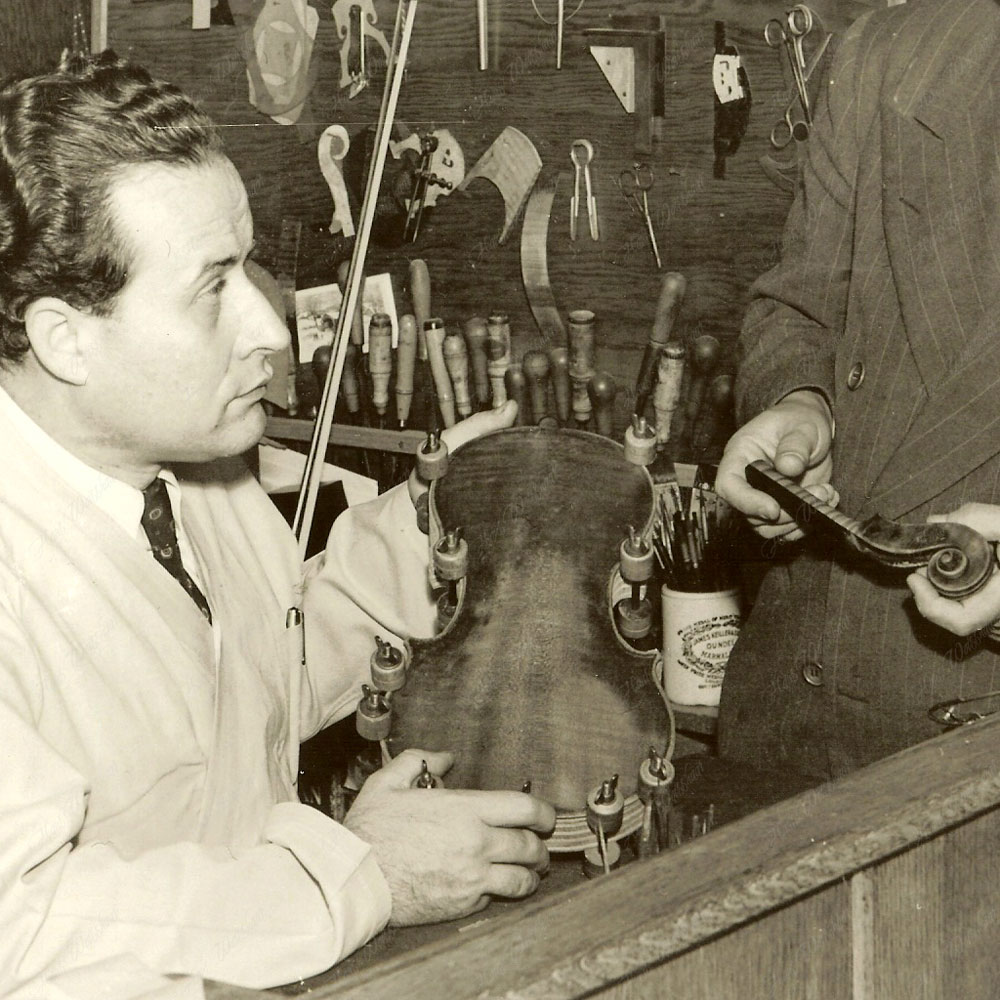In this detailed black-and-white photograph, two men appear to be in a dedicated violin repair or construction shop, surrounded by an assortment of tools and violin components hanging on the wall. The focal point is a man seated on the left, wearing a white coat over a patterned tie and white-collared shirt. He has dark, curly hair and a prominent nose, gazing toward the right side of the image. He holds the base of a violin, which is detached from its neck, indicating that it is in the midst of a repair process.

To the right, another figure, partially cut off from the image and only visible from his chest to his hands, stands holding the neck or scroll part of the violin. This second man is adorned in a dark pinstripe suit, and his head is not visible. The workshop setting is cluttered with a variety of specialized tools, files, and violin parts, hinting at a meticulous craft taking place. The combination of the men's focused expressions, the array of tools, and the segmented violin suggests a scene deeply rooted in traditional craftsmanship and musical instrument restoration.